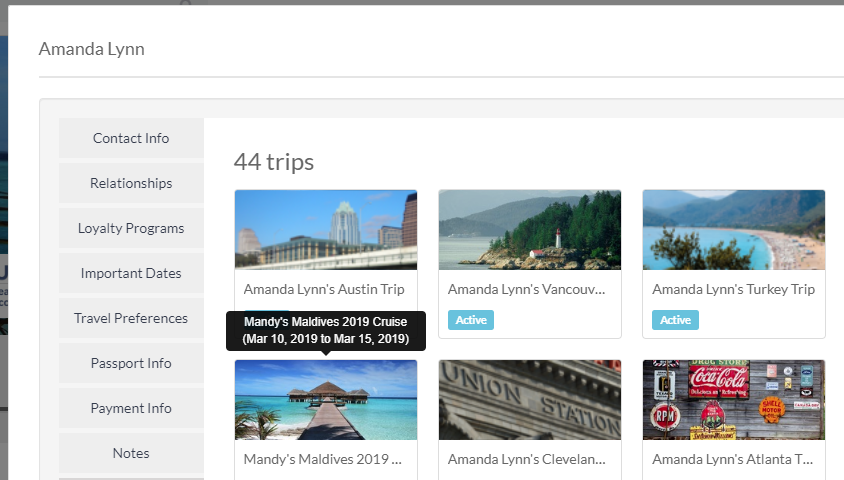The image is a screen capture of a travel management app or website displayed on a computer. In the upper left corner, the name "Amanda Lynn" is prominently written in black against a white background. Below this, a gray horizontal line separates the name from a vertical column of category buttons on the left side. These buttons list various categories for organizing information: "Contact Info," "Relationships," "Loyalty Programs," "Important Dates," "Travel Preferences," "Passport Info," "Payment Info," and "Notes."

To the right of this column, a section features a display of different vacation trips. It indicates a total of 44 trips, but only six are visible in the capture. 

The first trip on the upper left is labeled "Amanda Lynn's Austin trip," featuring an image of a city skyline. Adjacent to this, on the right, is "Amanda Lynn's Vancouver" with a picture of a lighthouse set against the scenic Pacific Northwest coast. Further to the right, "Amanda Lynn's Turkey trip" is showcased with an image of a sunny beach on the ocean.

In the bottom left corner, there is "Maddie's Maldives 2019," displaying idyllic ocean huts. To its right is "Amanda Lynn's Cleveland," with a picture of the historic Union Station building. Finally, on the far right, "Amanda Lynn's Atlanta" shows a wall adorned with an array of vintage gas station signs.

The meticulous organization and vivid imagery provide a comprehensive overview of the user’s travel experiences and preferences.